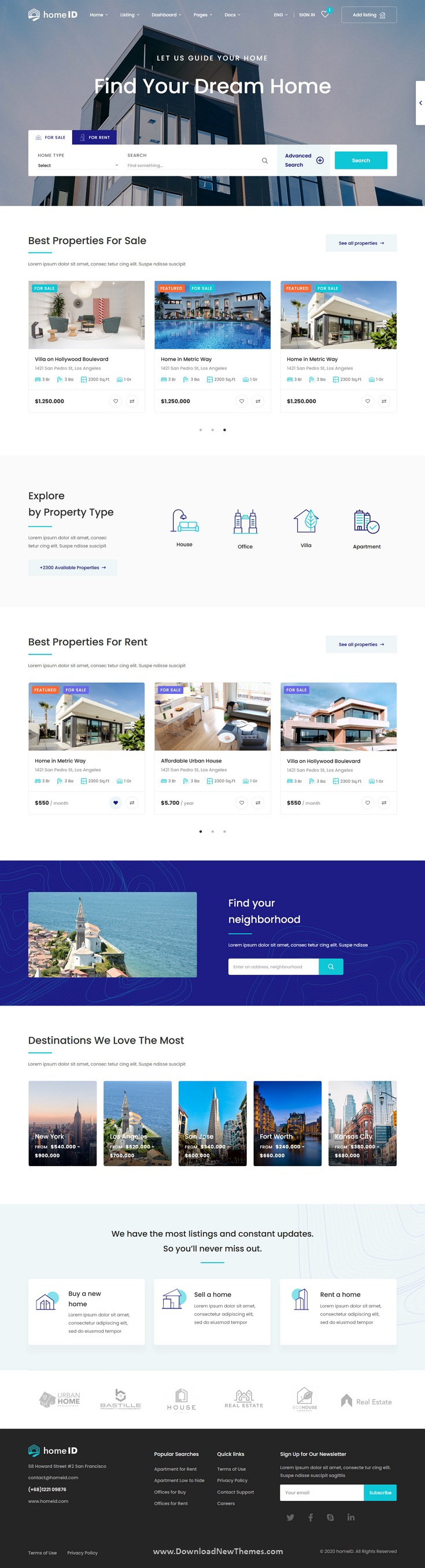This screenshot is from a phone and appears to be an online real estate listing website, though the small size of the image makes it difficult to identify the exact site. At the top of the page, there is a wide banner featuring an image with a grey background and a square building adorned with numerous windows. Overlaid text on this banner reads "Find Your Dream Home." Below this, there is a navigation bar colored white, with a blue accent at its end.

Further down, there are three horizontally aligned photographs. The first photo has a light-colored background, the middle photo features a dark blue water scene, and the third photo showcases a building structure. Each photograph includes a description and likely a price underneath.

Following this section, there is a grey strip running across the page. On the left side of the strip, there is some text, while to the right are four images arranged in a row. Below this, another section displays three more photographs. The first of these images shows a white roof extending over a building. The second image is ambiguous, resembling the interior of a house. The third image clearly depicts a large house with both a bottom floor and a partial top floor.